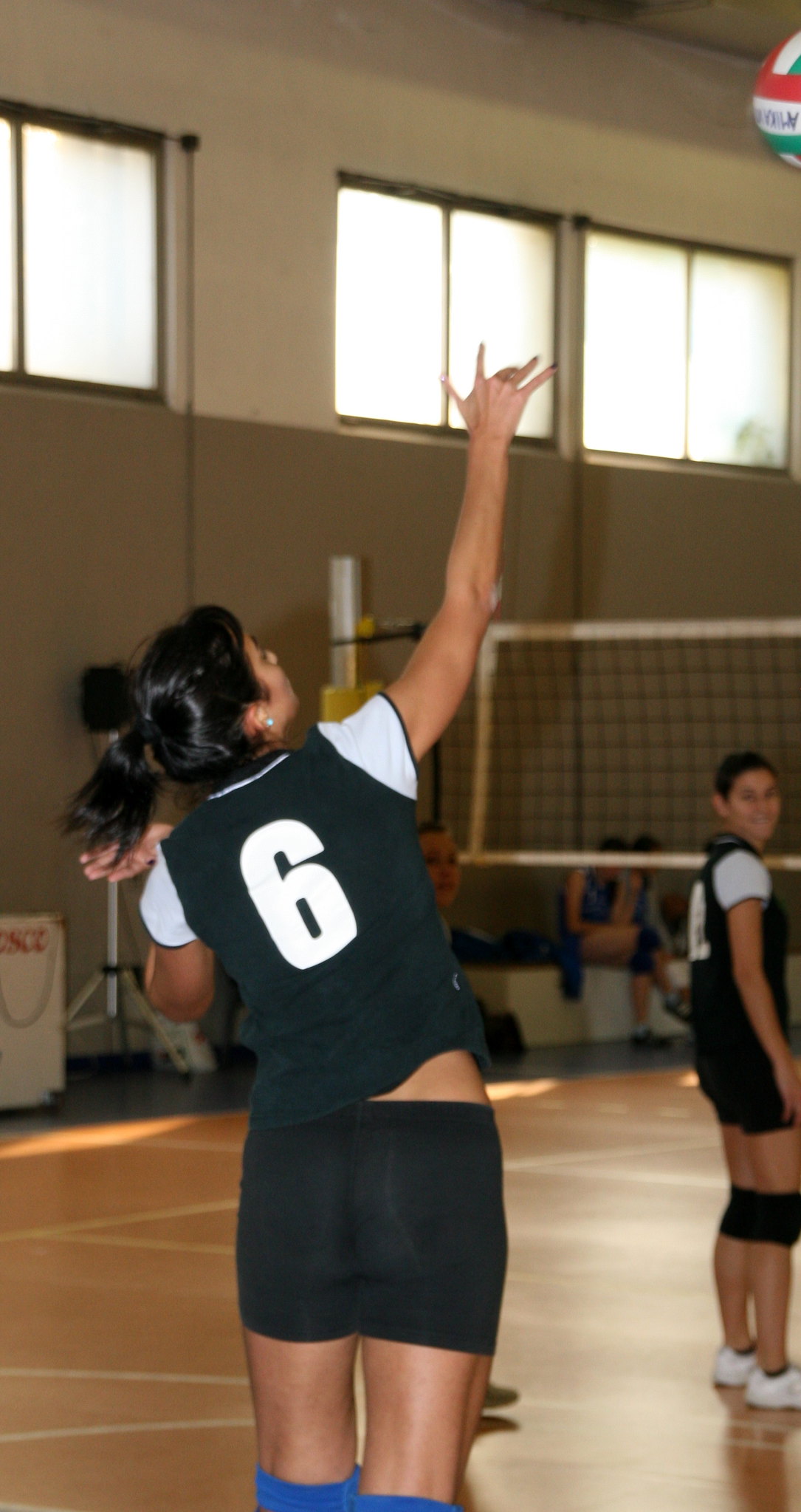The image is a vertical rectangular color photograph taken inside a gymnasium, possibly within a school, recreation center, or professional sports facility. The gym features a back wall that is dark gray on the lower half and light gray on the upper half, with large, black-framed windows allowing daylight to stream in, indicating it is daytime outside. 

In the foreground, the focus is on a volleyball game, primarily involving a women's team dressed in black uniforms with short white sleeves. At the center of the image is a woman wearing a black top with white sleeves, black shorts, and blue knee pads. She has glossy, black hair tied in a ponytail swinging to the left as she looks to the right with her right arm raised, having just hit the volleyball. The ball, which is white, red, and green, is captured in motion at the top right corner of the photo. The woman has a large white number six on her back.

To the right of the central figure, another teammate is partially visible, facing sideways and looking back at her. This teammate is also in a black shirt with white sleeves, black shorts, black knee pads, and white shoes. The volleyball net can be clearly seen stretching vertically about halfway up the right side of the image. In the background, a few people are seated on a bench along the side of the gym.

The opposing team is not clearly visible, but the overall atmosphere suggests an engaging moment of action during the volleyball game.